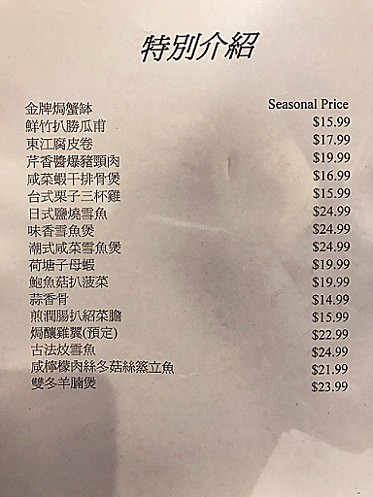The image depicts a close-up of a receipt against a plain background. The receipt itself is an off-white color and contains text in a foreign language. To the right, there is a column titled "Seasonal Price," listing the costs of various itemized purchases. The prices listed are as follows: $15.99, $17.99, $19.99, $16.99, $15.99, $24.99, another $24.99, and $19.99. The text detailing the origin of the receipt and the purchased items is prominently in a language other than English.